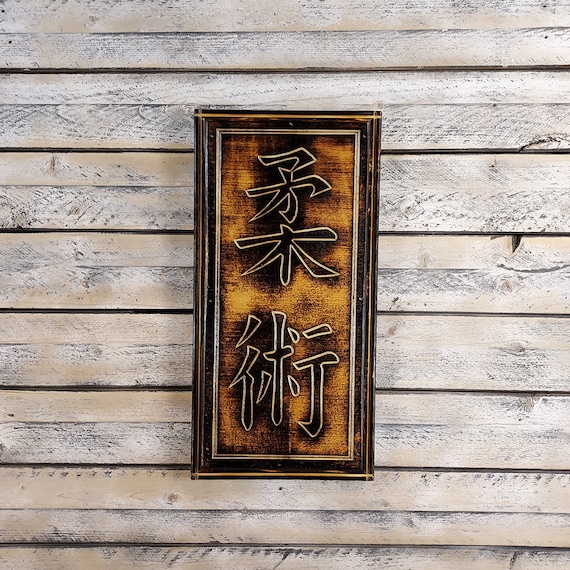The image captures a framed rendering, possibly of Japanese or Chinese characters, mounted on a weathered wooden wall composed of horizontal slats. The slats are lightly colored, almost blue-gray or beige due to natural weathering, resembling the side of a barn. The rectangular frame housing the characters is dark brown, and it stands out prominently against the aged wood. The characters or symbols, one positioned at the top and another at the bottom within the frame, are dark and possibly engraved or painted. The composition is well-lit, suggesting natural daylight, and the image is centered and slightly tilted, making the framed piece the clear focal point of the photograph. The colors in the image range from light to dark brown, beige, and hints of black, contributing to the rustic, natural aesthetic of the scene.